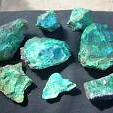This striking photographic image, presented in a small square format, captures eight turquoise to greenish-blue rocks meticulously arranged on a dark grey, almost black background. The scene is set indoors with no text distractions, allowing the varied textures and unique shapes of the rocks to be the focal point. The rocks are organized into three rows. In the bottom row, the first rock is a pointed, light green stone resembling a star, followed by a smaller, V-shaped rock, and a nearly rectangular stone. The second row features a blue-green rock with an oyster shell-like shape and a larger, spherical rock. The top row includes a triangular, almost blurb-like green rock, a smaller bluish pointed rock, and another similarly sized green rock. The arrangement appears deliberate, with shadows cast from a top-right light source enhancing the three-dimensionality and texture of the stones, further accentuating their unique forms and the subtle variations in their hues of turquoise and green.